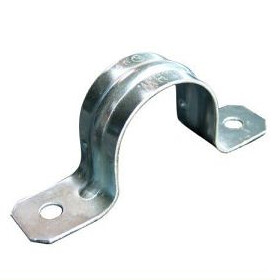This image depicts a silver metal handle, most likely made of sterling silver, placed against a plain white background with overhead lighting casting slight shadows. The handle starts with a flat segment on the left, ascends in a gentle arch, and then flattens out again on the right. Each end of the handle has a hole designed for screws or bolts, suggesting it can be securely attached to a surface such as wood or a wall. The object resembles an "N" shape with the arch rising in the middle, and it appears to feature some form of engraving on the top, although the details are indiscernible. The photograph captures the handle at a slight angle, enhancing its three-dimensional structure and highlighting its practical function as a tool or fastening device.